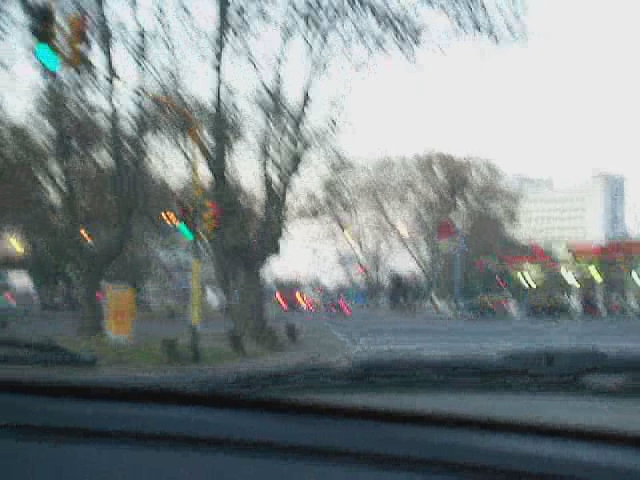The blurry image seems to be taken from inside a car, looking out through the front windshield onto a blend of vibrant colors ranging from white to green, yellow, red, blue, and pink. The bottom of the image includes a black windshield wiper and a gray surface likely representing the dashboard. Beyond the windshield, a gray-colored road stretches out ahead, flanked on the left by a dirt and grassy area dotted with brown wooden trunk trees and a yellow upward pole, possibly a streetlight or signpost. On the right side, there appears to be a gas station with a red roof and red signage, illuminated by yellow lights. Further back, several large buildings, other businesses, and streetlights can be discerned in the blurred landscape, along with a few cars on the highway. The sky is a mix of blue with white clouds, although its clarity is reduced by the blurriness, giving an overcast impression. The overall scene is indistinct due to the motion blur but retains enough detail to recognize these key elements.